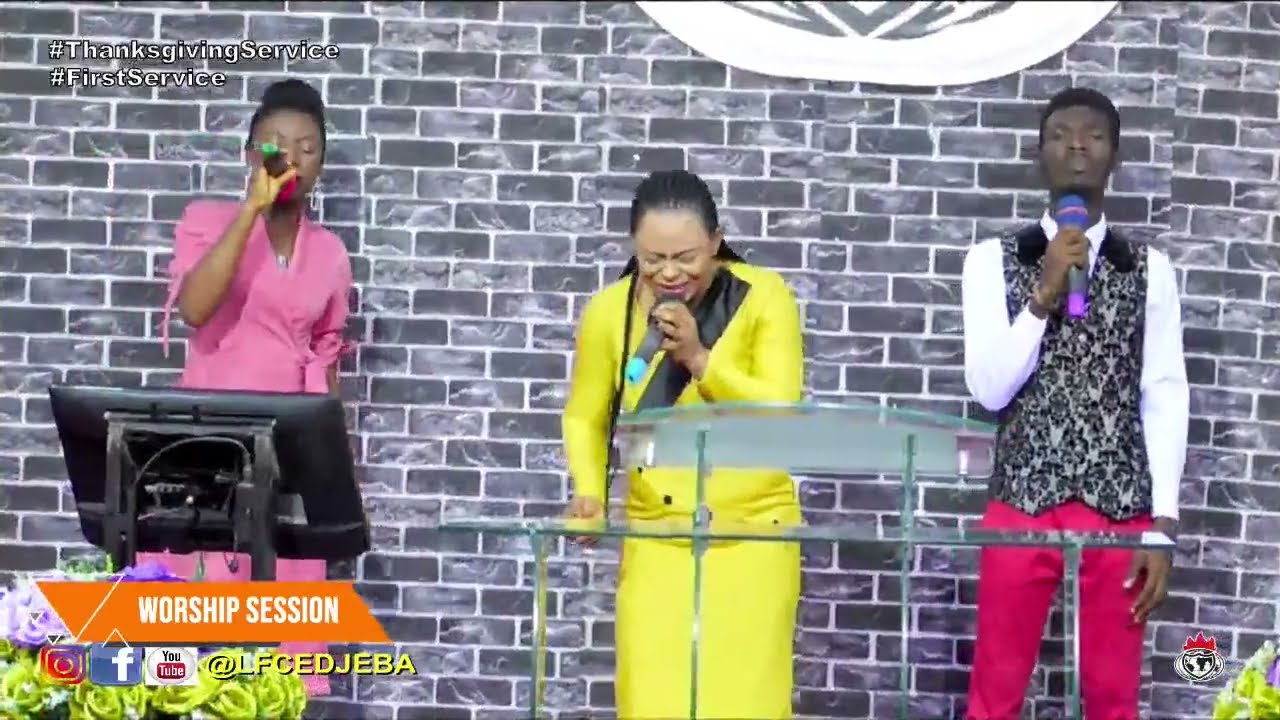This image captures a moment from a worship session, likely a Thanksgiving service, indicated by the hashtags "Thanksgiving Service" and "First Service" written in white in the upper left corner. The scene is set against a gray-toned brick wall and features a modern glass lectern with multiple panels and a curved top, likely used as a podium. The text "Worship Session" appears prominently in an orange bar in the lower left corner, accompanied by clickable social media logos for Instagram, Facebook, and YouTube, along with the handle "@LFCEDJEBA" in yellow writing that is somewhat hard to see.

Three African-American individuals are performing on stage. On the left, a woman dressed in pink passionately sings into her microphone. In the center, a woman stands confidently behind the glass lectern, dressed in bright neon yellow leather with a microphone in her hand. She has braided hair tied back and a black stripe running down the center of her outfit. To the right, a young man in red pants, a black paisley vest, and a white long-sleeved collared shirt holds a purple microphone at his chin, not currently singing. Behind them is a glass tabletop and there appears to be a computer monitor on the left side of the stage.